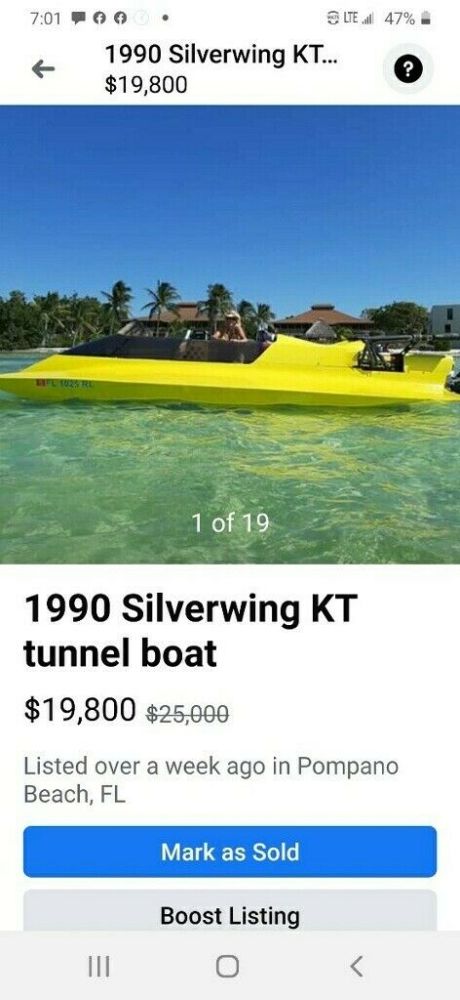A screenshot of a mobile device, likely an Android phone, displaying a for-sale listing for a 1990 Silverwing KT tunnel boat. The device's status bar at the top shows the time as 7:01, an LTE connection, and a battery level of 47%. The boat, now priced at $19,800 from an original $25,000, has been listed for over a week in Pompano Beach, Florida. The main image showcases a bright yellow boat floating on exceptionally clear, calm water, which is a striking blend of green and blue hues. In the background are picturesque palm trees under a clear blue sky. The presence of two buttons at the bottom of the screenshot—a blue button for marking the boat as sold and a gray button for boosting the listing—suggests that the screenshot was taken by the owner of the listing.